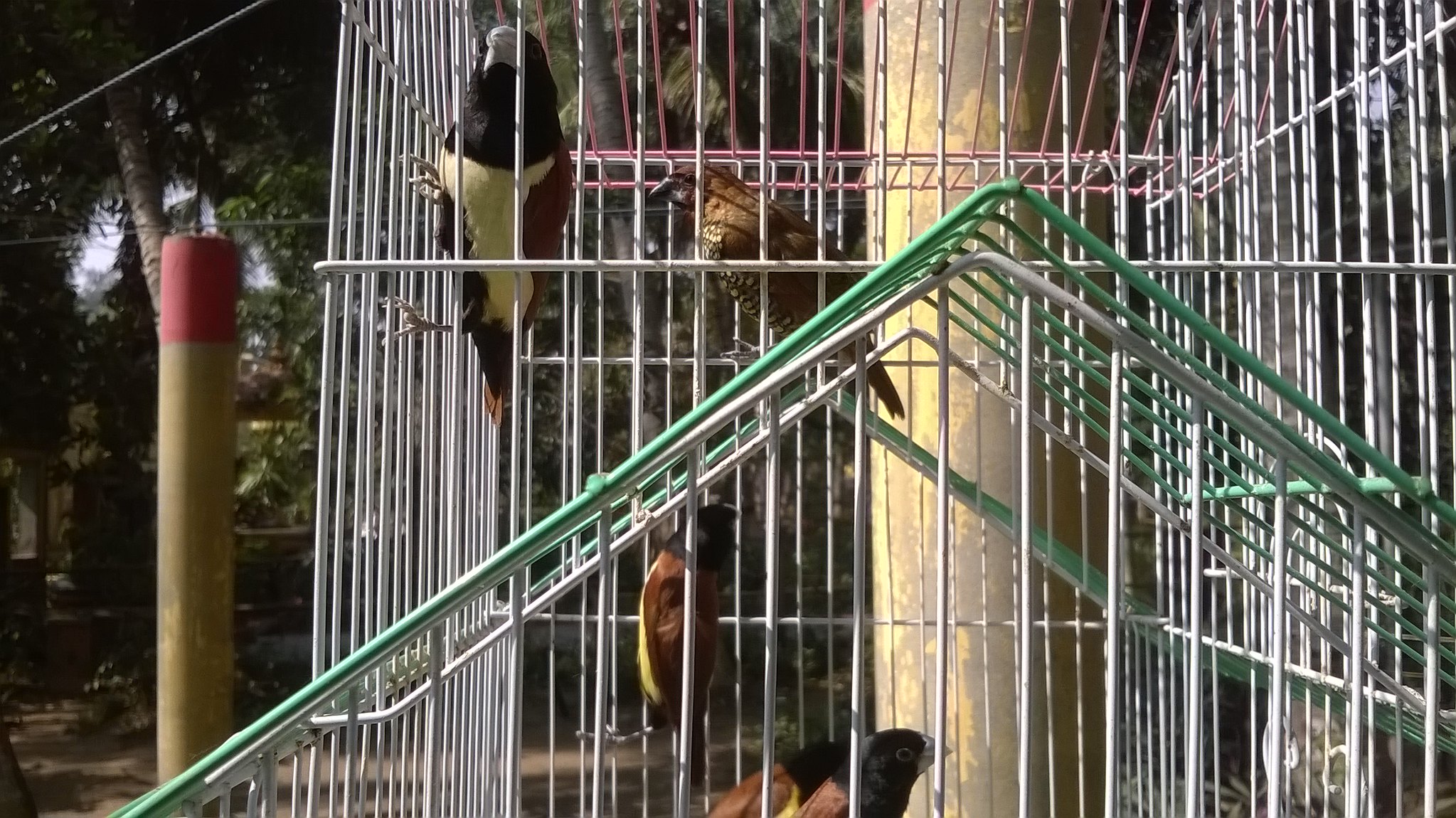The image features a central focus on two bird cages set against an outdoor backdrop, likely someone's yard. The ground surface appears to be a stone or concrete path, leading up to a dense background of trees, bushes, and grass. Positioned to the left of the image is a cylindrical pole with a greenish bottom and red top. Inside the prominently displayed white cages, there are several birds—counted to be around four to five. The birds display a variety of colors including yellow, white, and black. Notably, some birds have black heads and white chests, while others are predominantly yellow with black heads and some colorful beaks. The setting suggests a bright, sunny day with clear skies, as no rain is visible. Also, there is a mix of other colors such as green and pink from the wires of the cages.